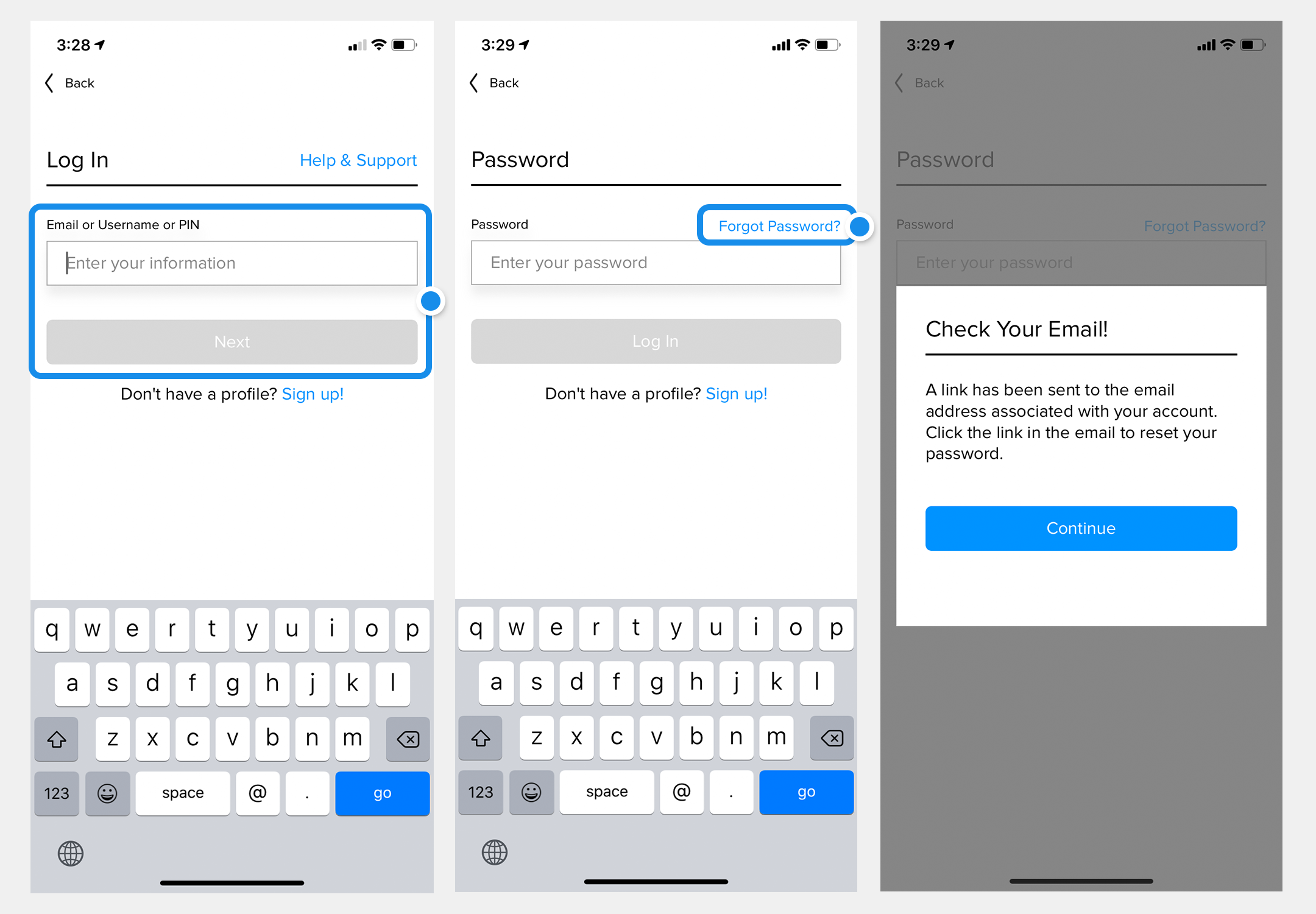This series of three split-screen images, displayed on an iPhone, illustrates the step-by-step process of resetting a password for an app.

**First Image (3:28 PM):** 
The screen displays the initial login interface of an app. At the top, the time is shown as 3:28 PM, accompanied by the Wi-Fi symbol and a half-full battery icon. The back button is visible, with "Log in" written to its right. On the far right, "Help and Support" is highlighted in blue. The main section prompts the user to enter their "Email or username or PIN" with a flashing typewriter cursor in a rectangular input field. Below this, a blue highlighted "Next" button is present. Beneath this button, a link reads "Don't have a profile? Sign up" in blue text. The bottom portion shows the user's keyboard in English.

**Second Image (3:29 PM):** 
One minute later, the screen now shows an interface for entering the password. The time updates to 3:29 PM. The back button from the previous screen remains, now accompanied by the word "Password." Users are prompted to enter their password in a designated input field. A small blue link, "Forgot password," is observable below the input field. The same blue "Log in" button is present, alongside the recurring "Don't have a profile? Sign up" link. The same English keyboard is visible at the bottom.

**Third Image (3:29 PM):** 
Still at 3:29 PM, this image likely captures the response to tapping "Forgot password." A white dialogue box with black text appears, instructing the user to "Check your email! A link has been sent to the email address associated with your account. Click the link in the email to reset your password." At the bottom of this dialogue box, a blue "Continue" button with white text is present.

**Overall Description:** 
The three images together form a tutorial on resetting a forgotten password within an unspecified app on an iPhone. Each step highlights the transition from logging in, to entering a password and eventually receiving instructions to reset it via email.